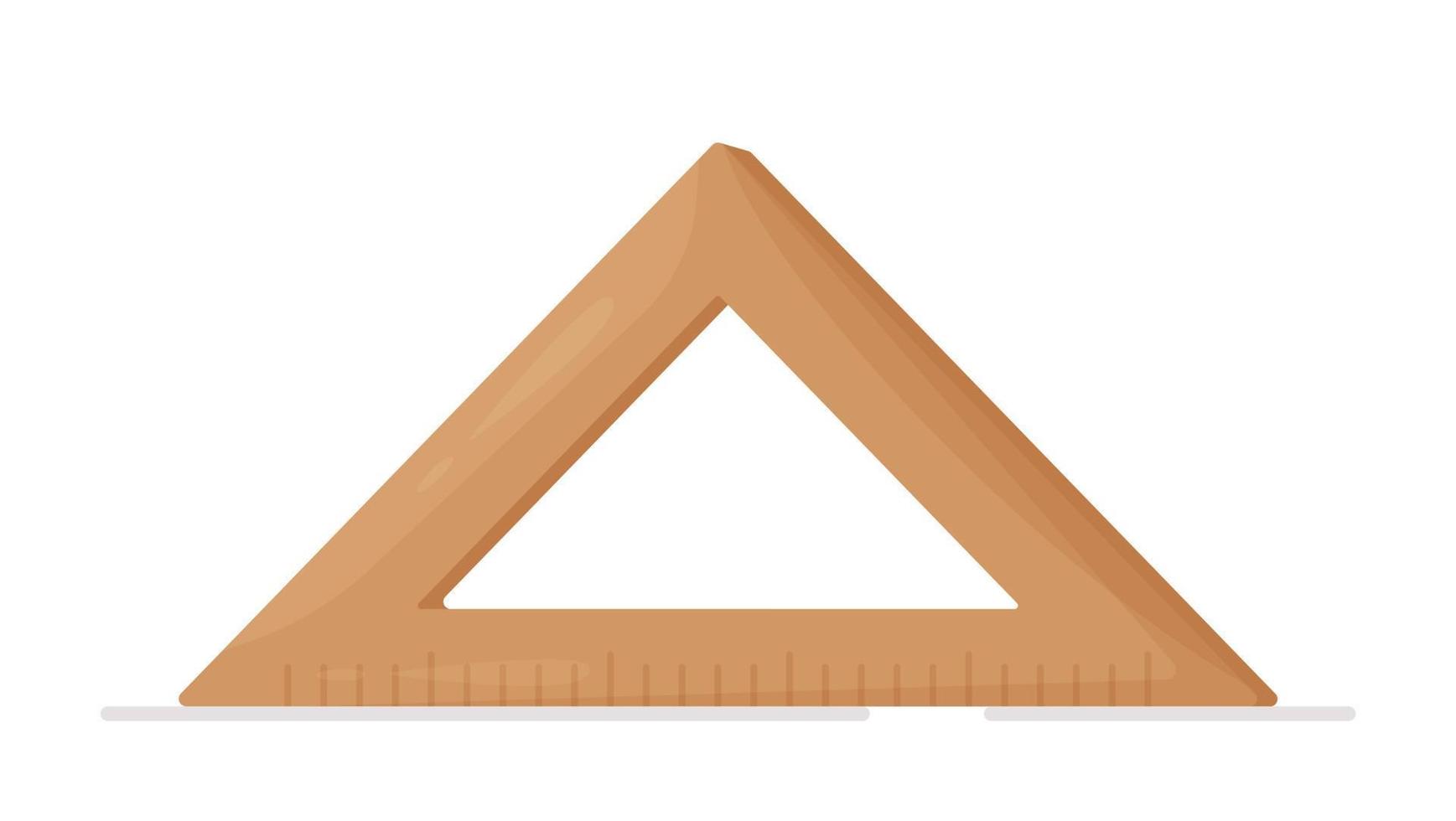The image depicts a digital rendering of a wooden triangular measurement tool, commonly used in drafting or architectural work. The triangle, which is light tan in color, features a right angle at its base and two acute angles at the top. The base of the triangle functions as a ruler, marked with notches to measure up to six inches. The triangle's interior is hollow, enhancing its resemblance to a technical drawing instrument. Rendered in a cartoonish, clip-art style, the tool stands out against a pure white background, emphasizing its intricate details and purpose. A subtle gray line beneath the triangle adds depth to the otherwise minimalist composition.